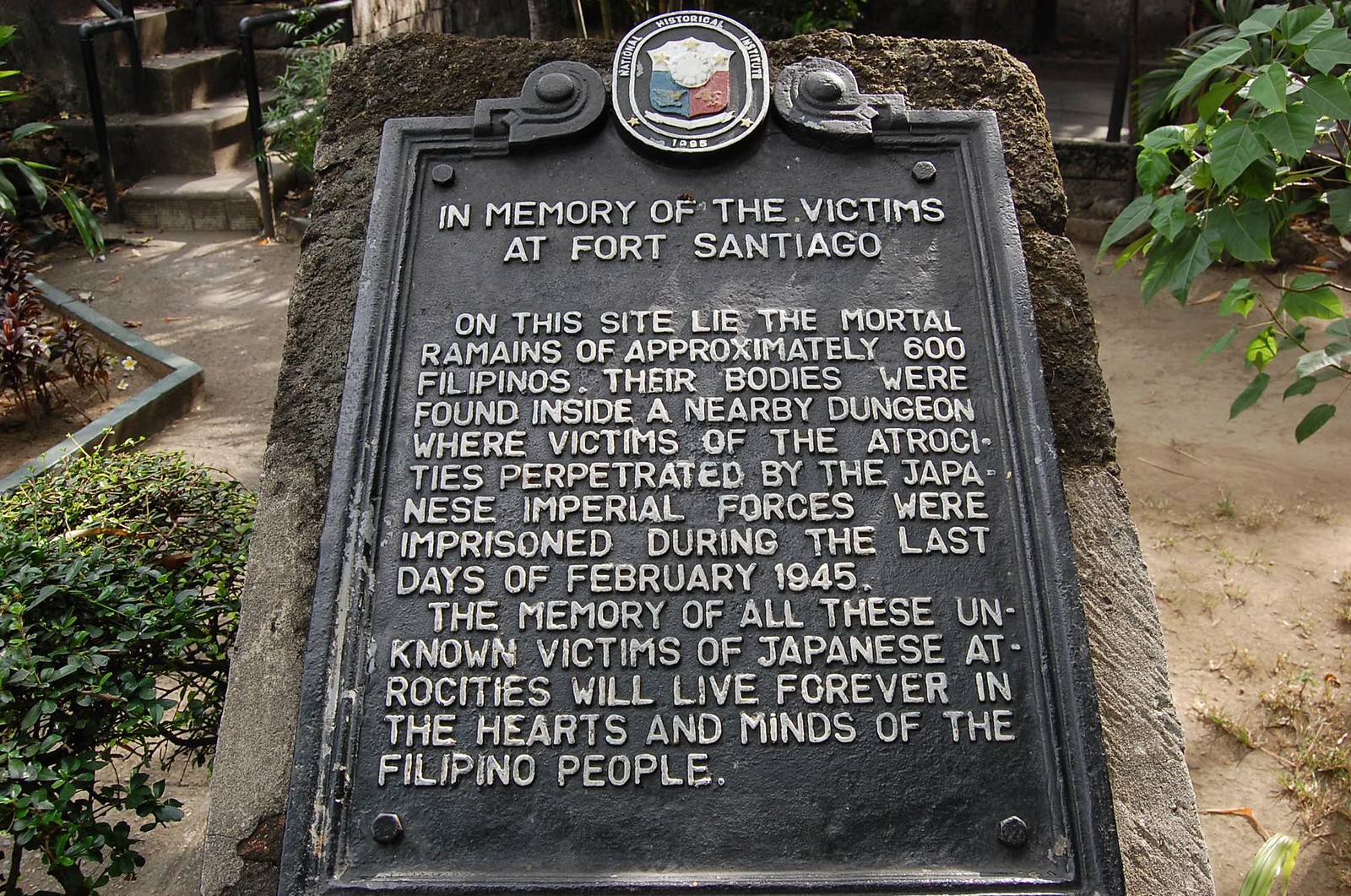The image depicts a solemn historical marker set in a garden area with a paved, concrete ground. At the forefront stands a large stone, tilted at about a 45-degree angle upward, bearing a metal plaque. The top of the plaque features a circular emblem with a red, white, and blue shield, and below it is an inscription that reads, "In memory of the victims at Fort Santiago." The plaque further details that on this site lie the mortal remains of approximately 600 Filipinos, whose bodies were discovered in a nearby dungeon where they were imprisoned by Japanese Imperial forces during the last days of February 1945. The inscription emphasizes that the memory of these unknown victims of Japanese atrocities will live forever in the hearts and minds of the Filipino people.

The stone itself shows signs of erosion, water damage, and possibly some moss, adding to its aged appearance. Surrounding the memorial, there are green leafy plants along the edges, and in the background, branches of trees and additional foliage can be seen. There are also stone steps with a handrail in the upper left and right corners of the image. The day appears to be sunny, with light filtering through the tree branches, casting a serene glow over the memorial site.